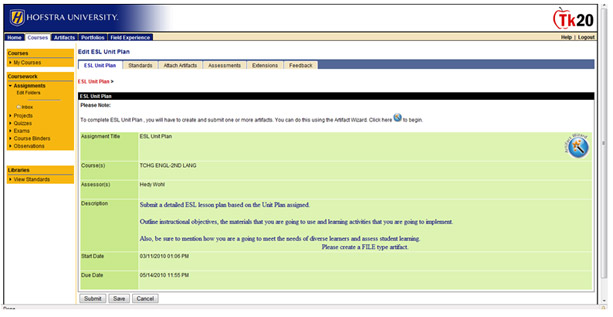This is an image of the Hofstra University website. The top left-hand corner features a shaded blue area. On the far left, there's an oval or teardrop shape with a yellow background and a sideways "H". Next to this, the text "Hofstra University" is written in blue.

Moving towards the right, the shading transitions from dark blue to light blue and finally to white at the far right side. An outline of an apple is also present, and inside the apple, the letters "TK" are in red while the number "20" is in black.

Continuing down the page, there are five dark blue tabs with white text. One tab is highlighted in white, labeled "Courses" in blue. Below this highlighted tab, there's a vertical orange rectangle that also says "Courses." Underneath, it reads "My Courses" with left and right-facing arrows on the left-hand side.

Further down, the text "Coursework" appears in black against an orange background. On the leftmost part of this section, a downward-facing black arrow is labeled "Assignments" in black text. The text "Exit Folder" follows in black.

Further down the left side, there's another right-facing arrow next to the text "Inbox" in black. Below this, there is another right-facing arrow next to the text "Projects." Moving further down, another right-facing arrow is next to the text "Quizzes." Underneath, another right-facing arrow is next to the word "Assignments" in black, and still another right-facing arrow next to the word "Exams." This pattern continues with arrows next to "Coursebinders" and "Observations."

Beneath these sections, there is a white horizontal rectangular bar for spacing. Underneath this bar, an orange horizontal rectangle is labeled "Libraries" in bold black letters. Below this, a gray horizontal stripe is visible. Finally, underneath the gray stripe on the left-hand side, there's a right-facing arrow next to the text "Few Standards."